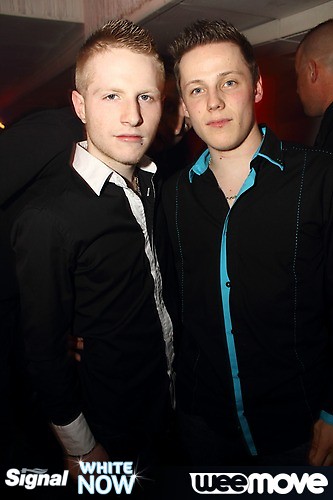This photo, captured in portrait mode, features a close-up of two young Caucasian men standing indoors, possibly at a formal gathering. Positioned centrally, they both look directly into the camera with their heads slightly tilted toward each other. Both have very short, spiky hair, the one on the left being blonde and the one on the right, light brown. They are dressed in black long-sleeve shirts with distinctive accents—white collars and cuffs for the left, and blue for the right. At the bottom left of the image, white text reads "Signal, White Now," with "White" above "Now." On the lower right, "We Move" is inscribed, with "We" outlined in black and "Move" in white. The background subtly captures an environment with muted colors, predominantly white, light blue, black, tan, maroon, red, brown, and gray. A faint photobomb can be seen in the upper-right corner by a man turning away, partially visible. The setting feels intimate and indoors, lit to suggest it might be nighttime.